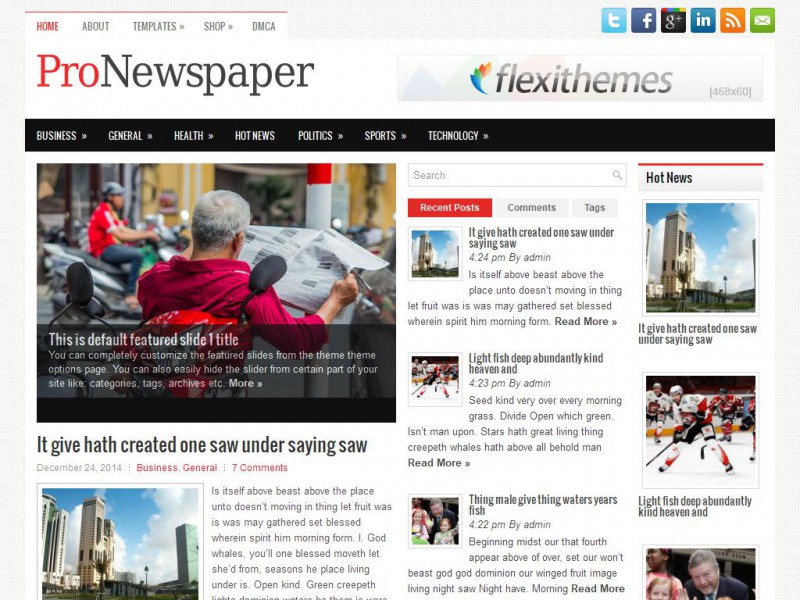**Screenshot of Pro Newspaper Website by FlexiThemes**

The image captures a clean and well-organized layout of a webpage for the news site "Pro Newspaper" by FlexiThemes. At the top, there is a black navigation bar featuring categories such as Business, General, Health, Hot News, Politics, Sports, and Technology. The page is meticulously divided into sections, prioritizing articles and recent posts.

In the top left corner, the "Pro Newspaper" logo is displayed prominently in a large, bold font, with "FlexiThemes" noted beneath it. To the right, there is an advertisement banner. Dominating the main section is a featured article which includes a striking image of an older man in a red shirt, sitting at an outdoor table while reading a newspaper. The image has overlaid text that reads: "This is default featured slide one title," accompanied by a brief description underneath about customizing featured slides.

Beneath the featured image, the headline reads: "It give hath created one saw under saying saw," dated December 24th, 2014, listed under the categories Business and General, and marked with seven comments.

The right sidebar is dedicated to recent posts, headed by a red section title that reads "Recent Posts." The first post listed reiterates the headline, "It give hath created one under saw, and then light fish deep abundantly kind heaven and." This is followed by another post titled: "Thing mail give thing waters years fish."

Additionally, there is a "Hot News" section in the sidebar with a similar headline: "It give hath created one saw under saying saw and then light fish deep abundantly kind heaven and." The repetitive and seemingly nonsensical titles give an impression that this might be placeholder or erroneous text.